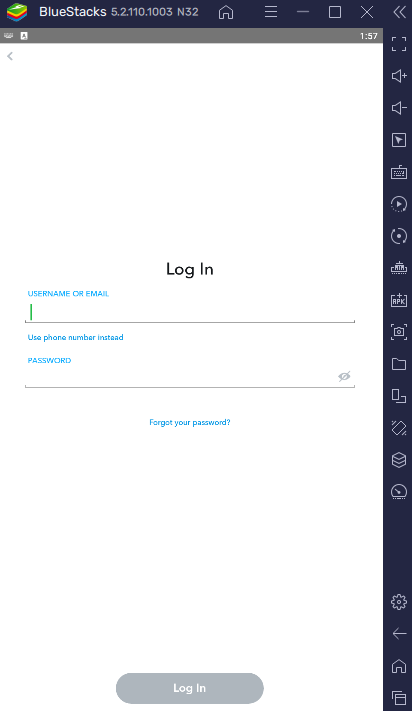This image depicts a side view of a mobile web page open on a smartphone. At the top, the header displays "BlueStacks" accompanied by a sequence of letters and numbers. Adjacent to the "BlueStacks" label is a small icon that looks like a stack of colored papers in the order of green, yellow, red, and blue.

The right side of the screen features a vertical, dark navy-blue rectangle containing various icons, each representing different functions. These include a speaker icon with a minus sign for volume down, a speaker icon with a plus sign for volume up, a video camera, a keyboard, a circle with rotating arrows for refresh, an icon depicting papers to indicate copying, and a clock symbol, among others.

In the central part of the screen, the page prompts users to log in. There is an input field highlighted with a green line where users can enter their username or email address. Below this, there is an option to "Use phone number instead" and a field for password entry. A link for "Forgot password" is also provided. Finally, a "Log in" button is prominently displayed at the bottom of the form.